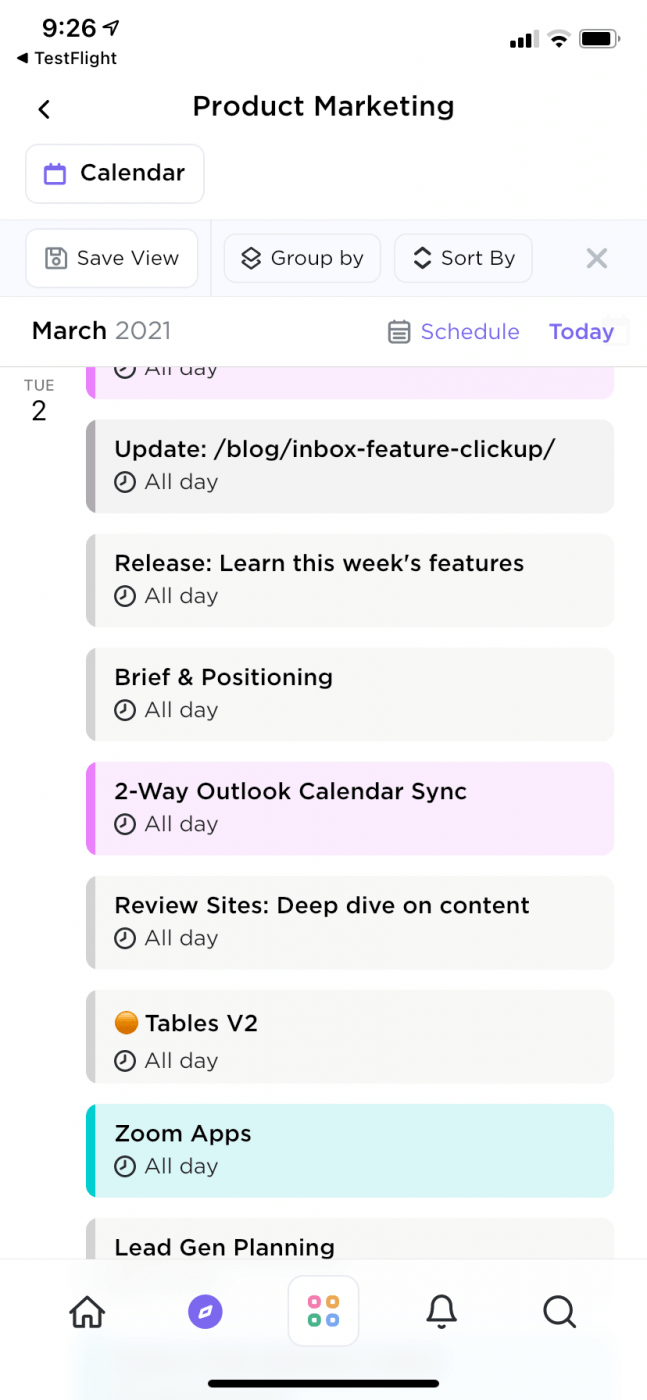Screenshot of a smartphone displaying the TestFlight app interface. At the top of the screen, the time is shown as 8:26, with an arrow pointing left next to the TestFlight label. The status indicators on the right include a strong signal and a full battery.

Below this, the screen shows the text "Product Marketing" against a white background. Underneath, there is a section labeled "Calendar" highlighted in a blue box. Continuing down, options such as "Save View," "Group By," "Sort By," and an 'X' button are displayed. 

The calendar section is for March 2021 and lists various scheduled tasks for Tuesday, the 2nd:
1. "Update Blog/Inbox Feature - ClickUp" (All day)
2. "Release - This Week’s Features" (All day)
3. "Brief and Position" (All day)
4. "Two-Way Outlook Calendar Sync" (All day)
5. "Review Sites - Deep Dive on Content" (All day)
6. "Tables B2" (All day)
7. "Zoom Apps" in a lime green box (All day)

At the bottom of the screen are icons for Home, Notifications, Search, Google, and the Phone app.

This comprehensive screenshot encapsulates a busy day filled with a variety of tasks and features, layered with a user-friendly interface for efficient schedule management.